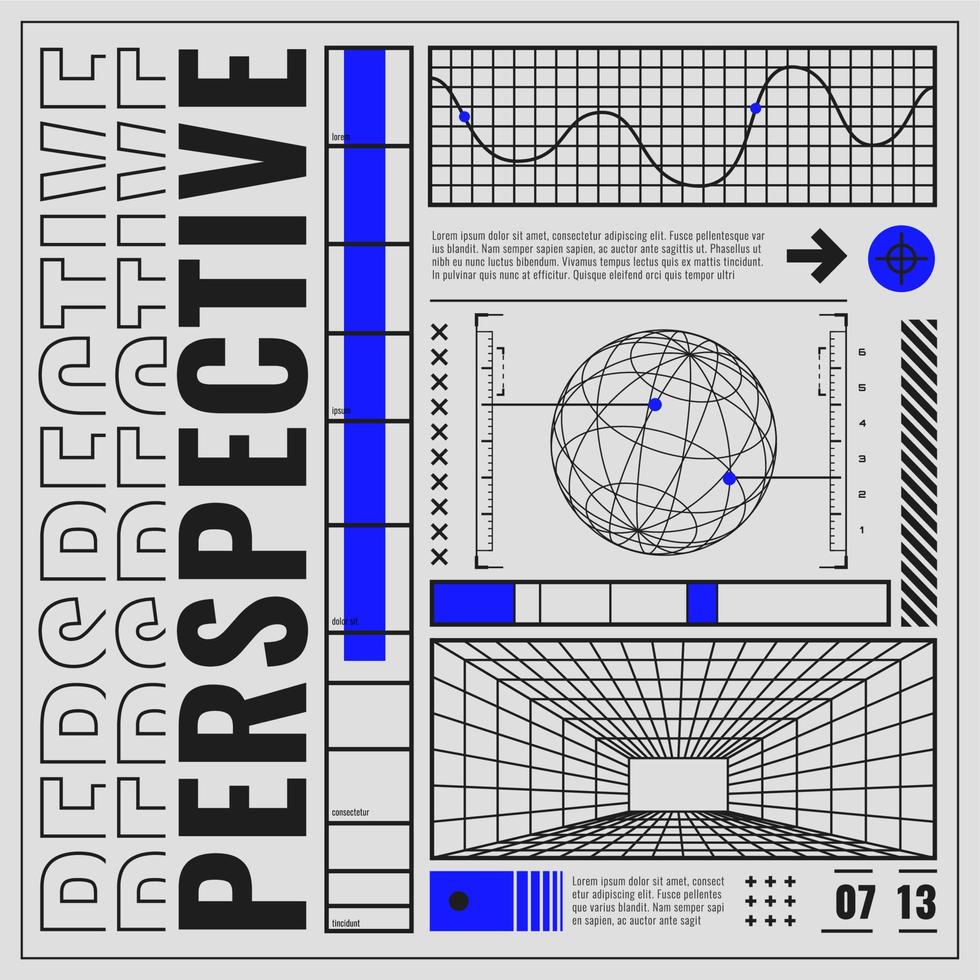The image is a detailed diagram with a light blue-gray background. Along the left side, vertically, the word "perspective" is bolded in dark black multiple times. The top half of the first two rows of this text is visible. Positioned centrally is a globe adorned with numerous intersecting lines, possibly representing a grid. Above the globe, there's a graph with illegible small print, highlighting intricate data lines. The lower portion of the image includes a 3D representation of a hallway, likely illustrating the concept of perspective in a visual and spatial context. Some areas of the diagram feature subtle blue lines and box-like structures enhancing the 3D effect, while the bottom displays the numbers "7" and "13."